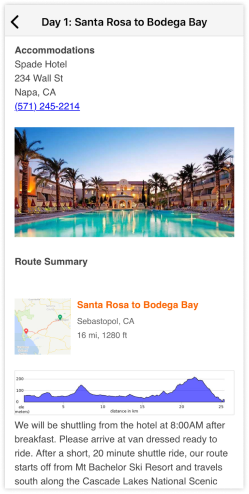**Day One of Vacation: From Santa Rosa to Batagor Bay**

Staying at the Spade Hotel on Wall Street in Napa, California, this vacation kicks off with stunning accommodations. The hotel features an enormous pool crowned by an array of tall pine, pineapple, and palm trees, creating an oasis-like setting enhanced by the surrounding hotel architecture. The pool area is extensive, comparable to the size of a football field, offering a serene and inviting atmosphere with its sparkling waters.

The journey from Santa Rosa to Batagor Bay covers a distance of 16 miles. Guests will gather at the hotel at 8 a.m. after enjoying breakfast, preparing for the day's adventure dressed and ready to ride. A short 20-minute shuttle ride will begin from the Mount Bachelor Ski Resort and head south along the scenic Cascade Lakes National Scenic Byway. This trip promises breathtaking landscapes and an exciting start to the vacation. Note that all guests must be prompt, assembling in the van by 8 a.m. to ensure a timely departure.